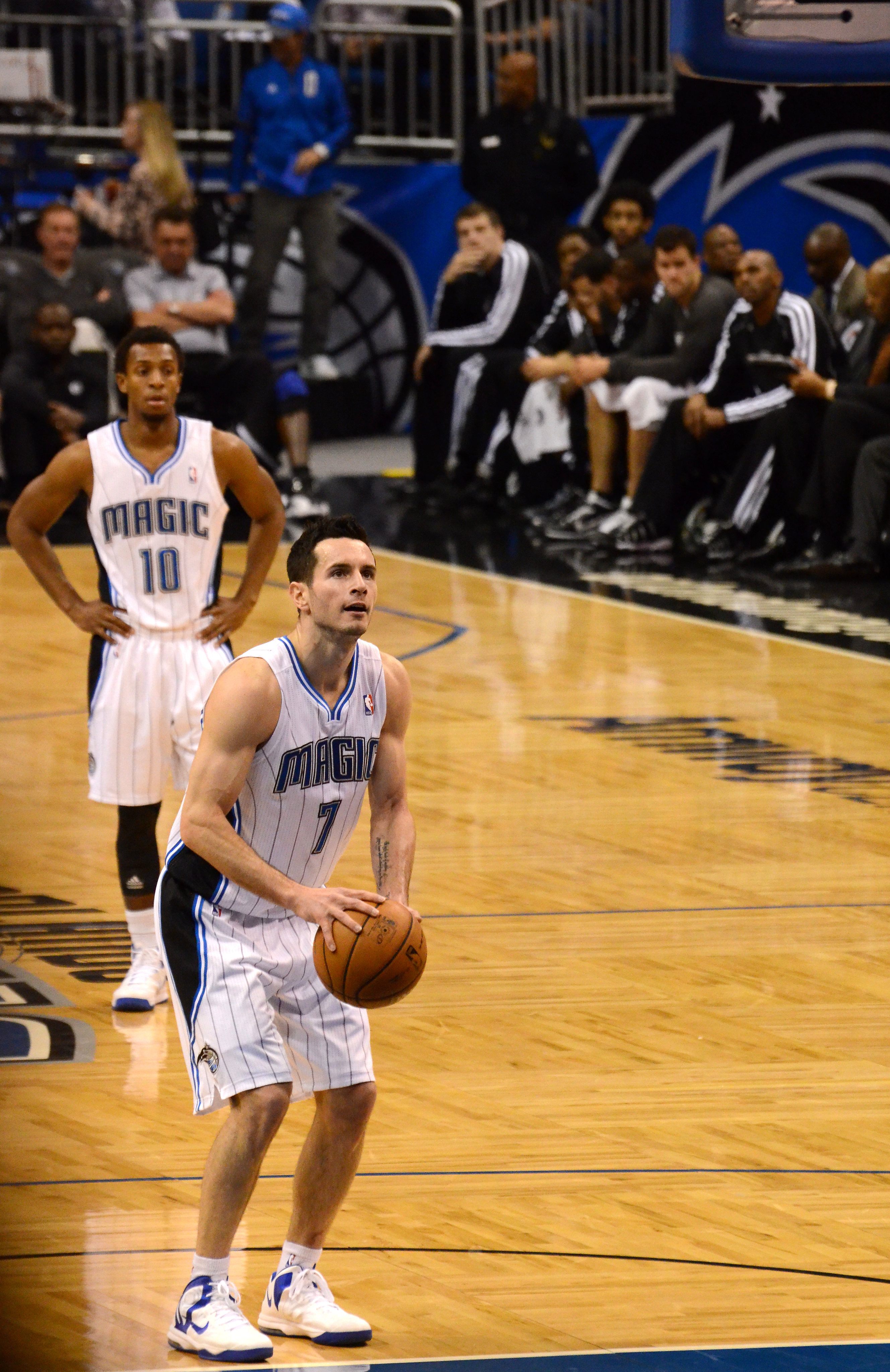The photograph captures an intense moment during an NBA game featuring the Orlando Magic. J.J. Reddick, in his distinctive white Orlando Magic jersey with black stripes on the sides and the word "Magic" in blue along with his number 7, stands at the free throw line, poised to take a shot. He holds the basketball with both hands near his hip, his knees slightly bent, clearly focused on the basket. Reddick's uniform is complemented by white and blue shoes and short white socks, and he sports a tattoo on his forearm and short dark hair. 

Just behind him stands another Magic player, number 10, watching the action with his hands on his hips. This player, a young black man with short dark hair, is positioned near the half court line, reinforcing the team's presence on the court. The gleaming wooden floor features a blue-painted area, including the free throw line and three-point arc, adding to the professional ambiance of the arena.

In the background, players of the opposing team, dressed in dark warm-up suits with white sleeves, sit on the bench, scrutinizing the free throw attempt. A security guard stands vigilantly, with scattered spectators seated slightly further back, all intently witnessing this fleeting yet significant moment in the game. The setting unmistakably reflects the home court of the Orlando Magic.